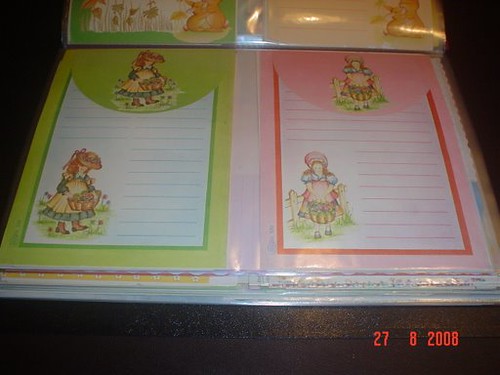This photo captures an assortment of stationery laid out on a very dark brown surface, possibly a desk, with a date "27-08-2008" in red letters in the bottom right corner, indicating when the picture was taken. The stationery is organized in a see-through flip file with plastic sleeves, opened to reveal two distinct yet similarly designed writing pads. The pad on the left features a lime green background with a central white block adorned with darker green writing lines. It also includes a repetitive illustration of a red-haired girl in a prairie dress with a smock, hat, boots, and a woven basket in the bottom left and top sections. The right pad mirrors this layout but in light red, featuring a different girl dressed in a pink smock with a bonnet and also holding a woven basket. The flash from the camera is visible, illuminating the scene and creating subtle reflections on the plastic sleeves amidst the otherwise dark setting.